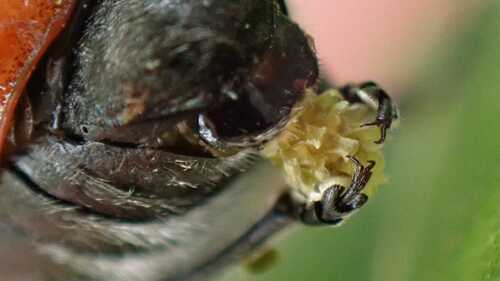This image is a highly detailed close-up of an insect with a black body and a reddish-orange exoskeleton. The insect is positioned almost straight-on with a slight tilt upwards. It is holding a small yellow flower with its segmented, tiny forked legs, appearing to chew on it. The legs are distinctly thin and segmented, showing precise detail. The background is heavily blurred, displaying a mix of green at the bottom and a creamy pink or peach towards the top. Additionally, the underside of the bug has a slightly furry white texture. The vivid colors, including green, yellow, black, reddish-orange, and white, stand out against the blurred outdoor setting, creating a striking contrast in the composition.